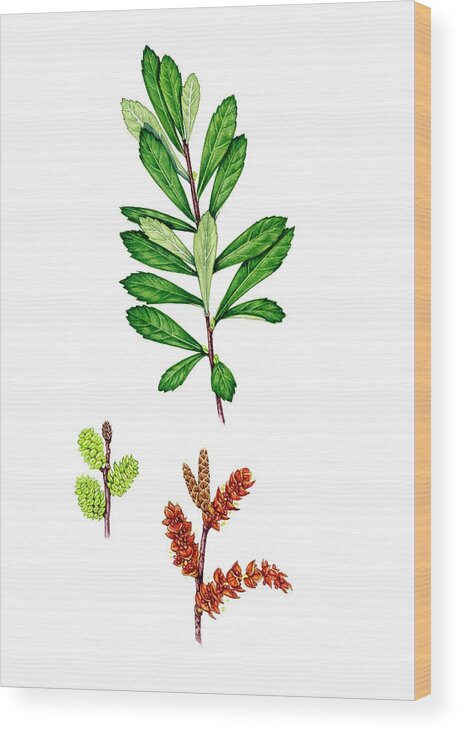This image is a depiction of a botanical artwork, possibly hand-drawn or digitally rendered, set on a vertical rectangular canvas with a textured off-white background. The canvas is bordered by a lighter tan, possibly wooden frame, which is only visible along the right edge, suggesting a sense of depth and thickness. Dominating the composition is a central sprig of green vegetation, featuring a main stem extending all the way to the top, adorned with variously sized green leaves, some dark and some light. Below this, toward the center-left, there is a plant with a purple stem bearing three prominent, oval-shaped green leaves that have a pinecone-like appearance. Finally, at the bottom center and extending slightly to the right, a third plant is showcased with a purple stem and bright red leaves or flowers, reminiscent of red chillies. This meticulously detailed artwork combines neutral and vibrant colors to create a visually appealing piece that would be suitable for display on a wall.